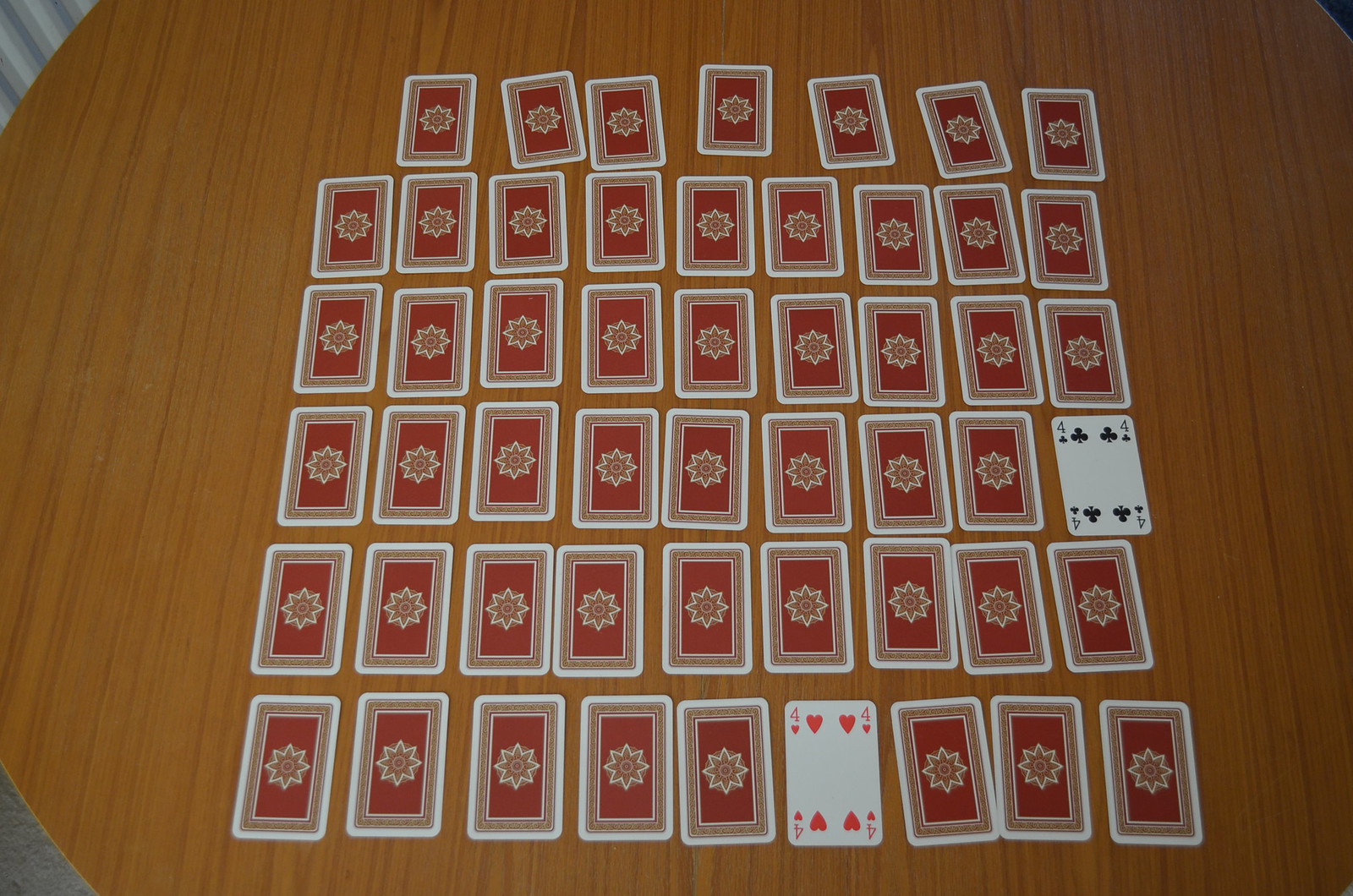In the foreground of the image, a collection of playing cards is displayed on a varnished wooden table. Among the cards, the four of hearts and the four of clubs are prominently facing up, their respective red and black suits visible. The cards are arranged in a grid-like pattern comprising six rows and nine columns, though the spacing is irregular, particularly in the top row where some cards are missing. The table's wood grain runs vertically through the scene, suggesting it is round in shape.

The decorative backs of the cards feature a red design, possibly floral or star-like, set against a white background with a detailed red and white border. This intricate pattern adds a touch of elegance to the otherwise casual setting of scattered playing cards. In the lower left and upper right corners, subtle shades of gray blend into the scene, adding depth and highlighting the natural patterns of the varnished surface.